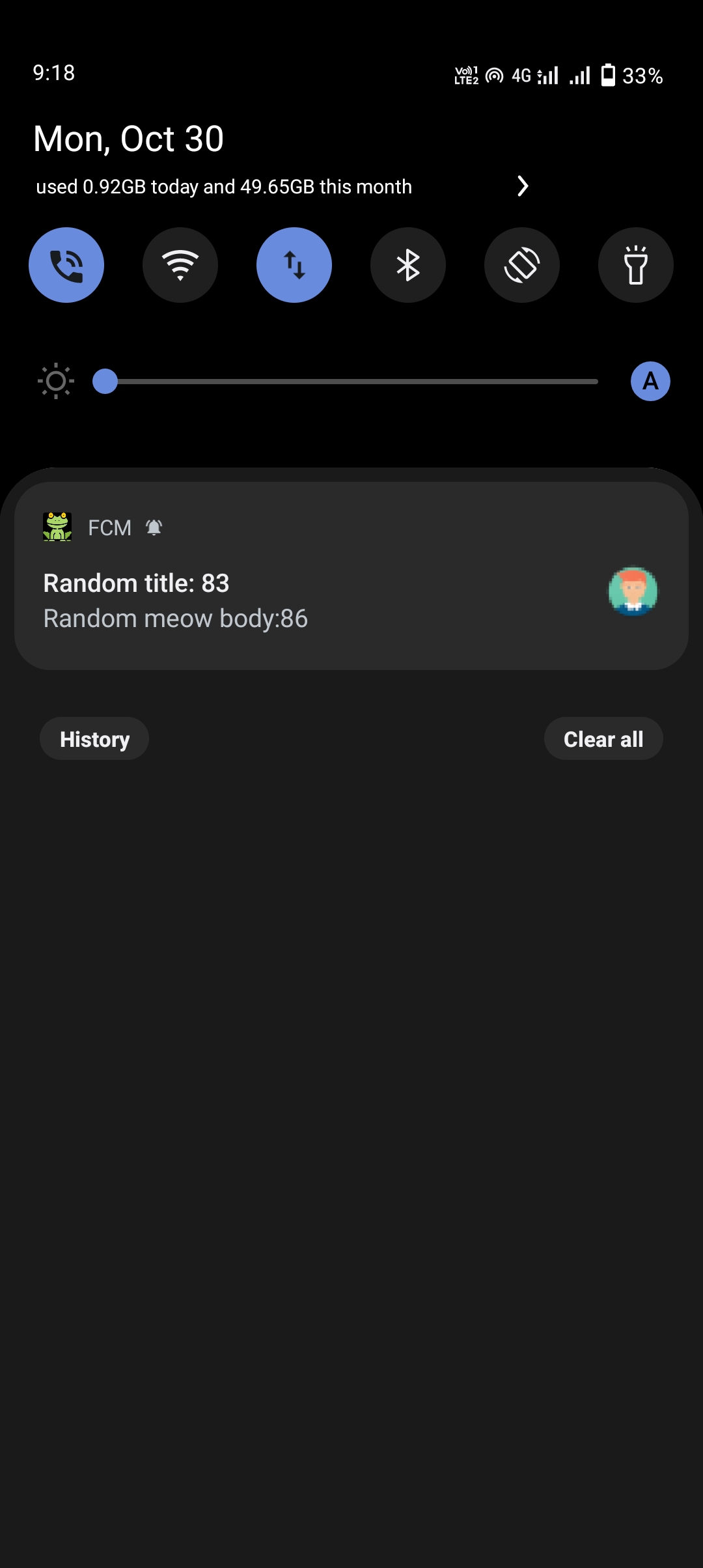This is a vertical screenshot primarily featuring black and dark gray tones. The top 30% of the screenshot is black, while the remaining 70% is a dark gray. It captures the screen of a smartphone. In the upper left-hand corner, the time displays as 9:18 AM. The upper right-hand corner contains various status icons, including a "4G" indicator, a Wi-Fi symbol, and a battery icon showing 33% charge.

Directly beneath this status bar, the date "Monday, October 30th" is displayed. The screen also informs the user that they have used 0.92 gigabytes of data today and 49.65 gigabytes this month.

Further down, there's a section with various icons. A blue phone icon appears first, followed by a grayed-out Wi-Fi symbol indicating that Wi-Fi is off. Next, a blue icon with arrows pointing up and down appears, representing data transfer. This is followed by a gray Bluetooth symbol, a grayed-out vibrate icon, and finally, a gray flashlight icon.

A brightness slider is positioned below these icons, currently set all the way to the left (minimum brightness). Adjacent to the slider, on the right, is a blue "ace" symbol.

The notification section below this displays a message from FCM with the title "random title 83" and the body "random meow body 86." The notification includes a small icon of a man with orange hair. Beneath the notification, there are two buttons: "History" on the left and "Clear All" on the right.